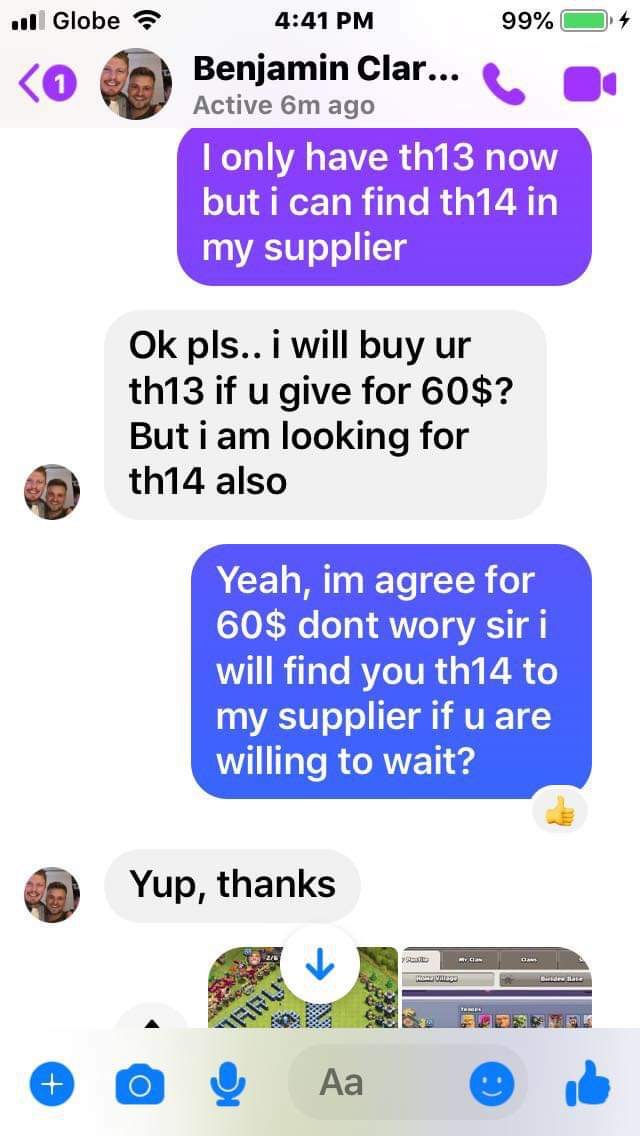This image is a detailed screenshot from a cell phone depicting a conversation on a messaging app, likely Facebook Messenger, as indicated by the style and layout. At the top of the screen, the status bar shows a strong signal strength, a full Wi-Fi icon, the time (4:41 PM), and a nearly full battery at 99%. The conversation is with a contact named "Benjamin C-L-A-R..." who was active six minutes prior. 

The text exchange reveals the sender discussing the availability of items labeled TH13 and TH14 with Benjamin. Initially, the sender informs Benjamin, "I only have TH13 now, but I can find the TH14 with my supplier." Benjamin responds, "Okay, please... I will buy your TH13 for $60, but I am looking for TH14 also." The sender agrees to the price, replying, "Yeah, I'm agreed for $60. Don't worry, sir, I will find you TH14 from my supplier if you are willing to wait?" To which Benjamin concludes with, "Yep, thanks."

The text bubbles are color-coded, with the sender's messages highlighted in blue and Benjamin's in white, a typical feature in Messenger apps to distinguish between the two participants.